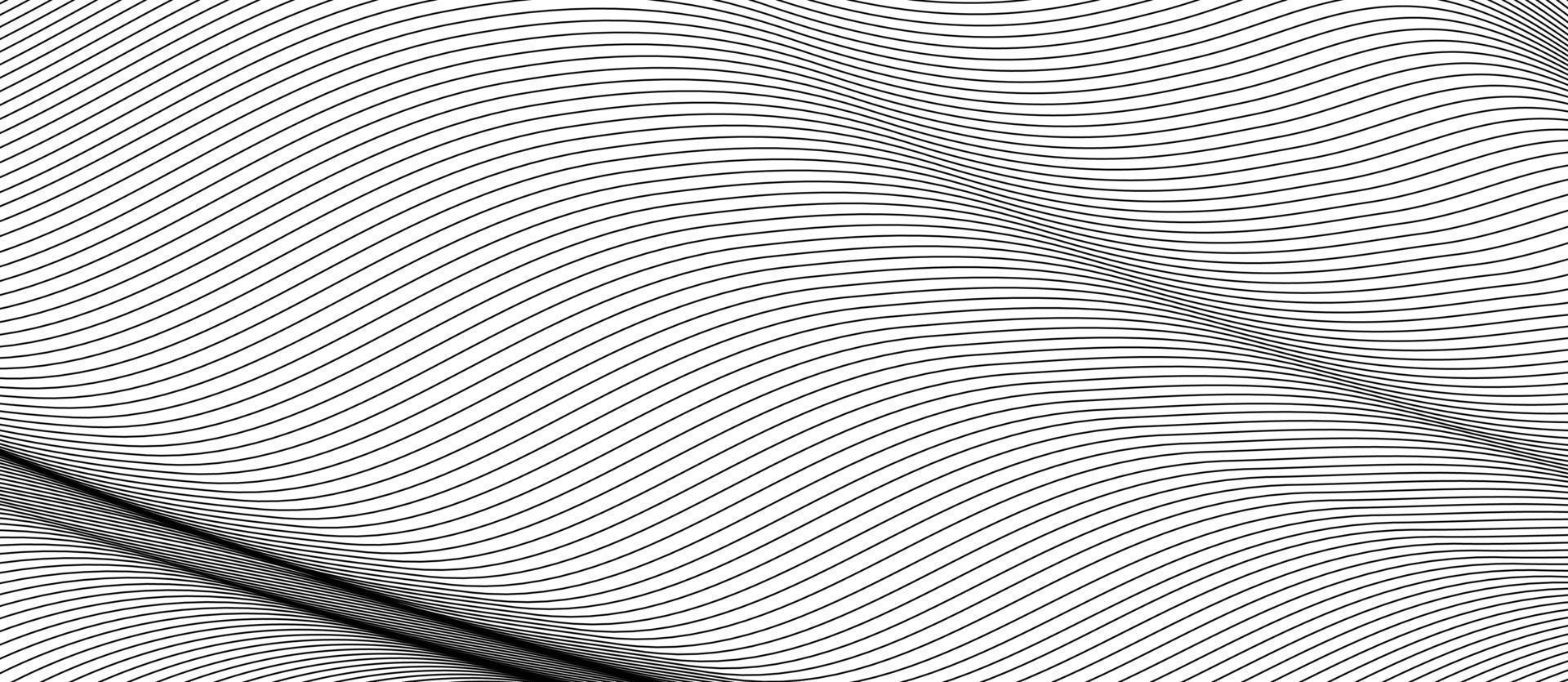The image depicts a horizontally long and vertically short pattern of narrow black lines on a white background. These lines undulate in a wave-like fashion, creating an optical illusion of motion. The lines vary in amplitude from gentle to pronounced waves, extending diagonally across the image. In the bottom left corner, a pair of darker lines intersect the waves, adding depth and dimension to the design. The intricate pattern of narrow lines, approximately a millimeter or two in width, combined with the shadowing effects in some areas, evokes a sense of swirling and movement, almost as though the fabric-like lines might fold or crease. The overall effect is a mesmerizing blend of geometry and illusion that captivates the viewer's gaze.